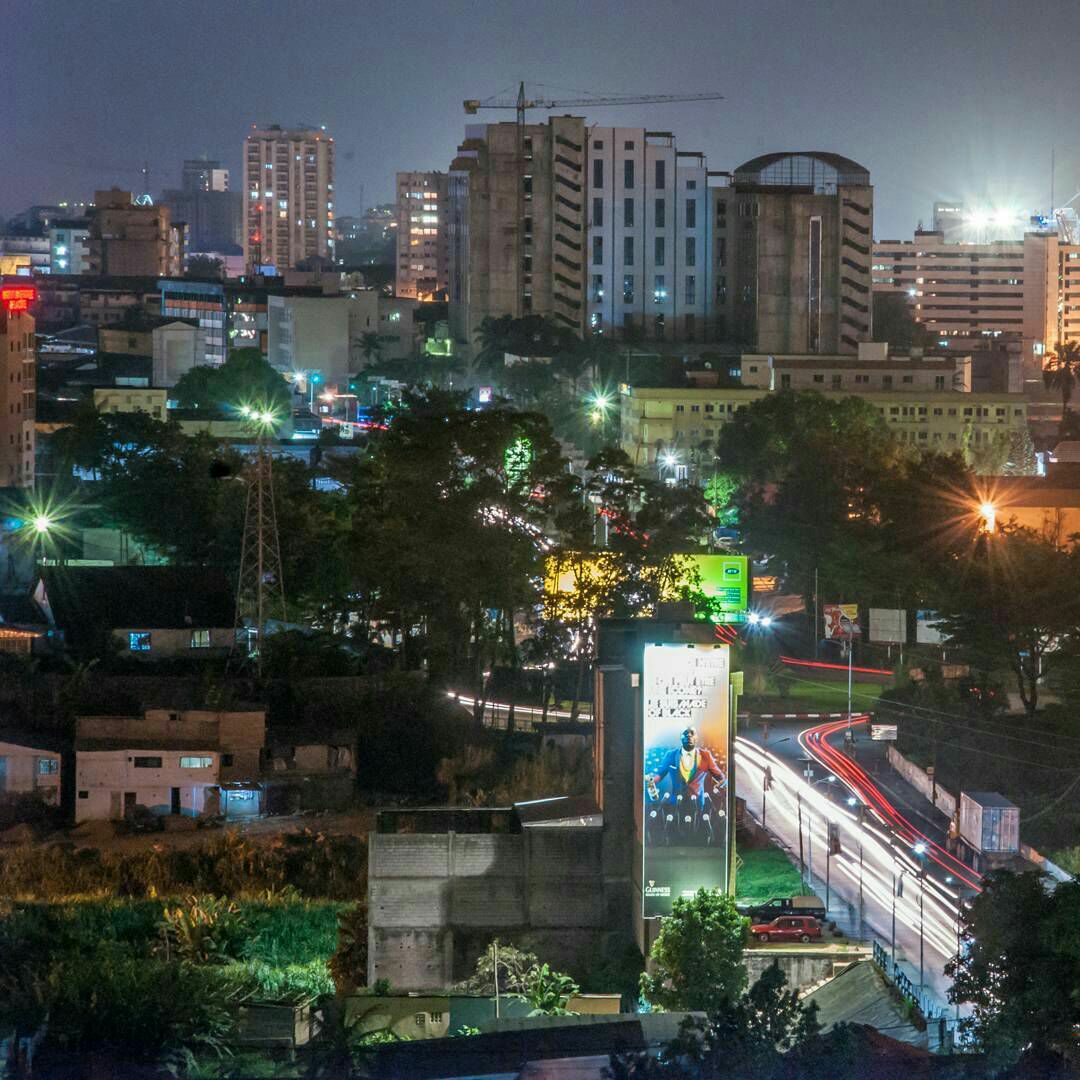This nighttime, time-lapse photograph captures the bustling cityscape of Douala, Liberia, showcasing its impressive blend of urban infrastructure and natural elements. Dominating the scene are numerous high-rise skyscrapers, their windows aglow with lights, painting a vibrant picture against the bluish-gray, light-polluted night sky. The city appears alive and active, with streets radiating under street lights and headlights, creating streaky red and white lines of moving traffic. In the foreground, a prominent roundabout acts as a hub of activity, bordered by various buildings. A notable illuminated billboard featuring a gentleman stands out, alongside other neon signs and advertisements. Amidst the concrete structures, patches of greenery and trees intersperse, adding a natural contrast to the urban environment. A construction crane towers above one of the buildings, indicating ongoing development. Additional details include a semi-truck hauling cargo along a highway, a parking lot with a red car and a dark truck, and graffiti on a retaining wall. The photogenic clarity and scenic beauty make this a captivating snapshot of Douala's nighttime allure.